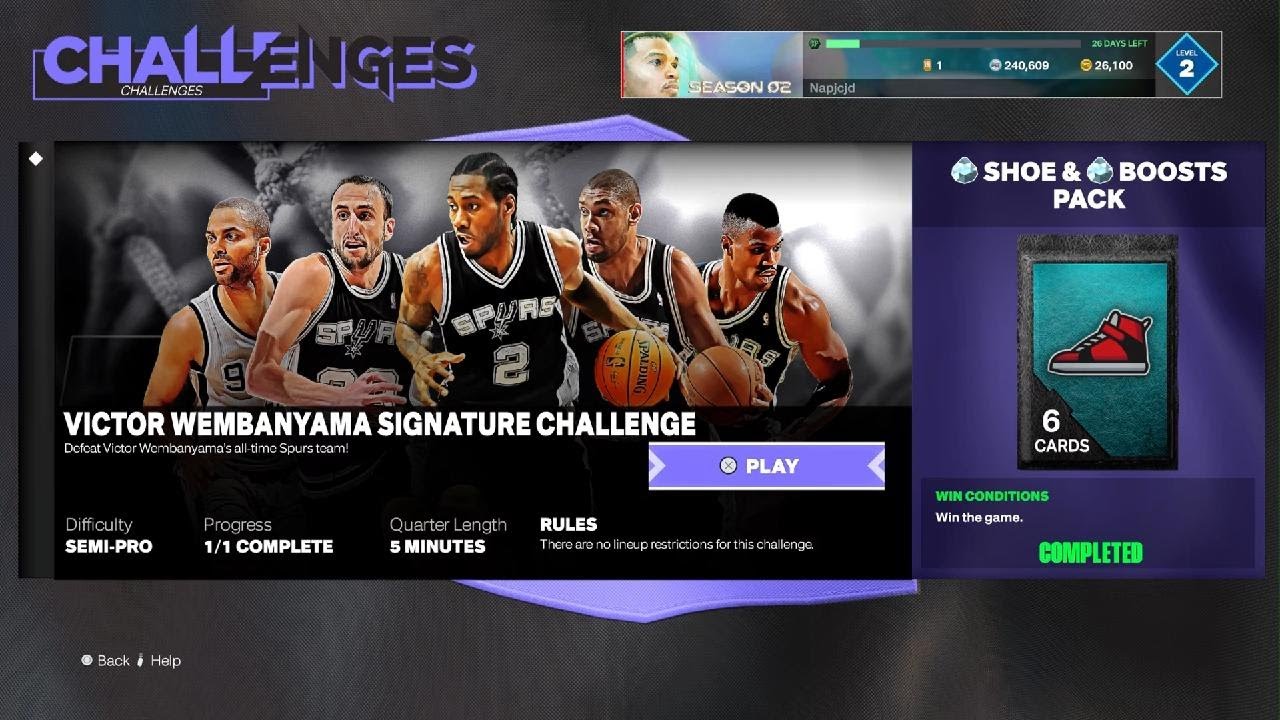The image features a rectangular layout set against a black background. At the top of the image, the title "Challenges" appears in a unique font that is partly purple and partly black, making the black portions difficult to see. To the right of this title, a slender rectangle showcases a person named Deacon Oz, displaying his face. Adjacent to this is another rectangle with unclear text except for a prominent diamond shape containing the number two.

The central focus of the image is a group of five basketball players wearing Spurs jerseys. This section is overlaid with text that reads "The Victor Wenbenyama Signature Challenge," presented in a slightly transparent black rectangle to stand out against the background.

Further details include a purple rectangle with the word "Play" written on it and a bottom line that states "Semipro 1/1 complete," along with "five minutes and rules." On the far right, there is a card featuring a red sneaker, labeled "Shoe Boost Pack" and indicating the inclusion of six cards. The word "Completed" appears in green, suggesting the challenge has been successfully finished.